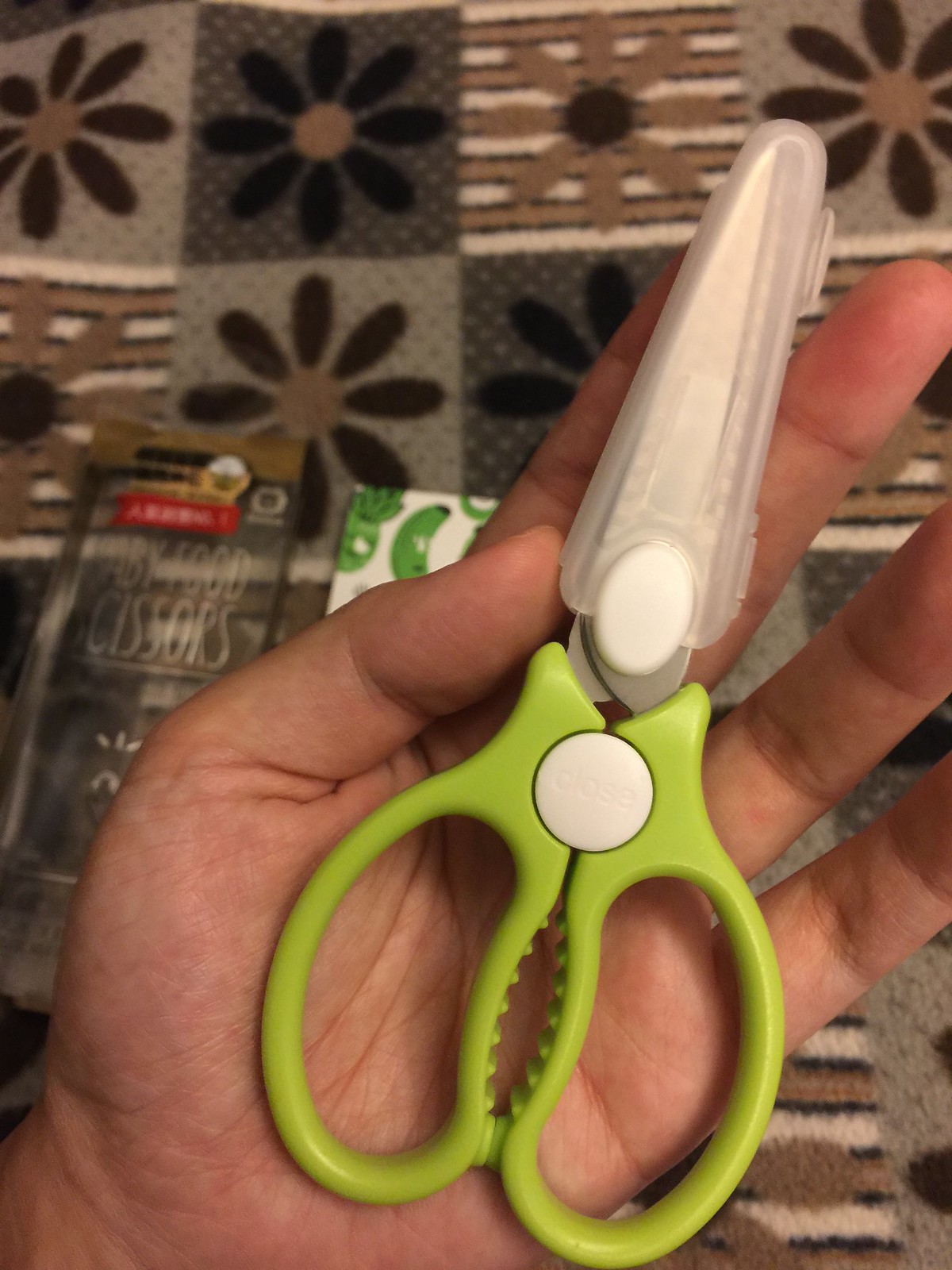The photograph shows a close-up of a person's left hand, prominently displaying a small pair of green-handled scissors, which are likely designed for craft or baby food purposes. The person's palm cradles the scissors, clearly revealing the hand's relatively young appearance. The scissors feature a bright green plastic handle with two white buttons at the hinge, and the short, matte metallic blades are sheathed in a clear plastic protector for safety. Encapsulated in the handle is a small round tablet labeled "Close." The background showcases a quilt with a busy floral pattern in hues of black, gray, light brown, dark brown, and olive green, organized in a checkerboard fashion. Partially visible on the quilt is the packaging for the scissors, labeled "baby food scissors," and an obscured booklet with green illustrations.